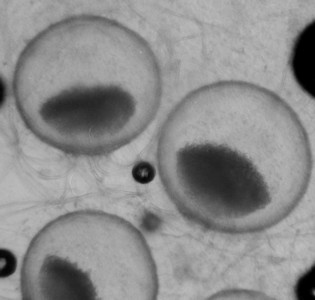This black and white, perfectly square image presents a microscopic view of cells. The primary focus is on three clear, circular spheroid cells, each associated with distinct structural details. Located in the upper left-hand corner and center-right are two prominent spheroid cells, enclosed within faint tissue or fiber-like background. The cells exhibit gray patches inside and are each tethered to an oval-shaped black circle with a white center. At the bottom of the image, partially cut off by the edge, is another spheroid structure. Scattered throughout the background are various smaller and larger black circles, further adding to the intricate details of the cellular composition. The image is devoid of text, human figures, and color, emphasizing a purely scientific visual of cellular structures under high magnification.